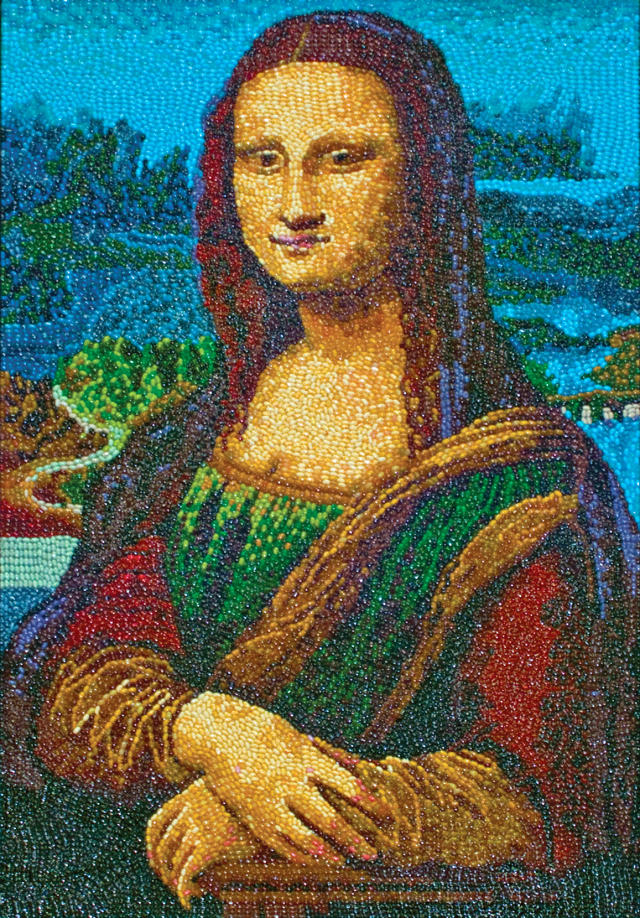This is a vertical rectangular image showcasing a modern adaptation of the Mona Lisa, rendered with incredible intricacy, resembling beadwork. The background features a dynamic blue palette with varying shades, including dark and light blues, alongside green elements that suggest the presence of bushes. Mona Lisa herself stands out with her long, dark hair and signature enigmatic smile. She is depicted in striking, colorful robes: green crosses her chest, a yellow cape adorned with green drapes over her shoulders, red accents mark the upper part of her sleeves, while yellow decorates the lower sleeves. Both her hands are visible and rest on what appears to be the wooden arm of a chair, distinguished by a white stripe.

Upon closer inspection, the image conveys the appearance of being composed entirely of tiny seed beads, adding a textured, tactile quality. The beads create a spectrum of colors: her hair, intriguingly, seems to incorporate shades of red, purple, and black, while her skin glows with golden and yellow hues. Her attire is a blend of yellow, gold, green, blue, black, red, and camel colors, all meticulously placed to form a vibrant and detailed representation. The beadwork expands into the background, where the blues and greens blend seamlessly, possibly indicating the ocean and surrounding trees. This carefully crafted, visually stunning image of the Mona Lisa reflects both modern artistic techniques and a nod to classical iconography.